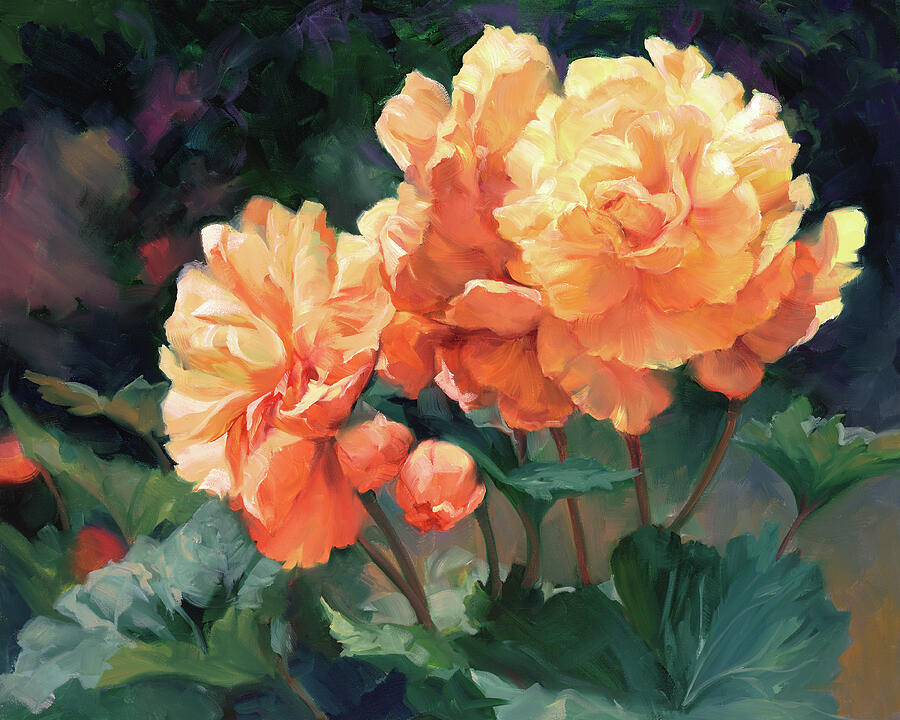The painting depicts a delicate bouquet of vibrant yellow-orange flowers, glistening under light. Prominently, three fully bloomed flowers are clustered at the center, with an additional two smaller, unopened buds to the left. The flowers are surrounded by large, verdant green leaves, emanating from individual stems. The background is a rich tapestry of dark greens with splashes of pinks and hints of beige, providing a fuzzy, vegetative contrast. Subtle purple hues intermix among the leaves and stems, enhancing the depth and layering of the scene. The flowers, bathed in sunlight, exude a bright and lively energy, capturing the essence of nature's delicacy and vibrancy.